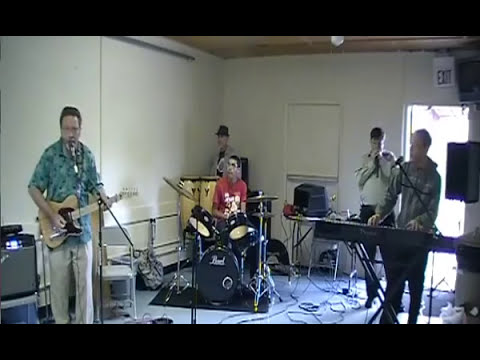The image depicts a band performing or rehearsing in a white-walled room with a lot of ambient light entering through an open door on the right side, highlighting the exit sign above. The room features a large whiteboard or projector screen to the left, behind which several black cords and amps are scattered on the smooth, gray floor. The band consists of five members: on the far left is a man with a brown and black guitar, wearing a green button-down shirt and khaki pants. In the center, one man in a red shirt plays black drums, while another in a tan shirt and top hat is positioned behind him, likely playing hand drums such as bongos or conga drums. To the right, a man in a green hoodie and black pants plays a black keyboard, and behind him is another man in a white hoodie holding a microphone to his mouth. Additionally, a mat lies under the drums, and a gray chair is placed behind the man singing. The scene is framed by black strips at the top and bottom, emphasizing the indoor, possibly garage-like setting of the band’s rehearsal or performance.